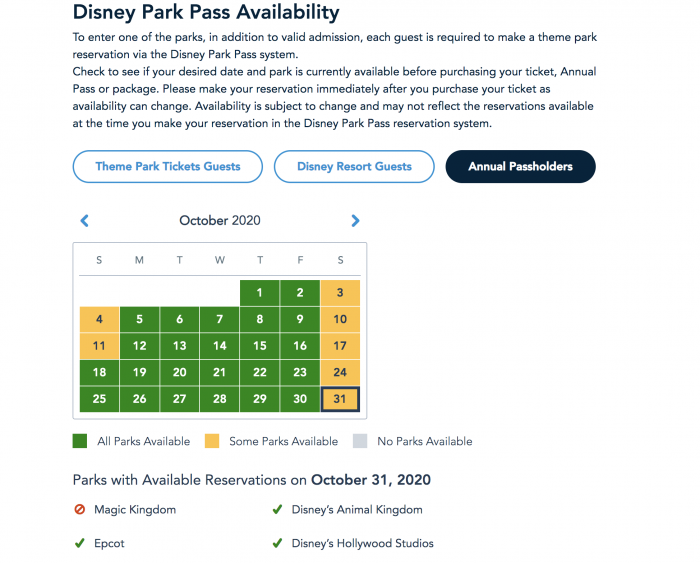This image, captured from a phone or iPad screen, displays the "Disney Park Pass Availability" page. To access any of the Disney parks, guests need a valid admission along with a mandatory theme park reservation via the Disney Park Pass system. It's crucial to check the availability of your desired date and park before purchasing tickets, an annual pass, or a package. The image advises making your reservation immediately after purchasing a ticket, as availability can change rapidly. The page includes three clickable sections tailored for different types of guests: "Theme Park Tickets Guests," "Disney Resort Guests," and "Annual Pass Holders."

At the center of the image is a calendar set to October 2020. Below the calendar, a color-coded key indicates the reservation status: green signifies all parks are available, yellow denotes that only some parks are available, and gray means no parks are available. The calendar highlights that most Saturdays and Sundays show alternating availability with some parks open and others not.

Specifically for October 31, 2020, the parks with available reservations include Epcot, Disney's Animal Kingdom, and Disney's Hollywood Studios. However, Magic Kingdom is fully booked and unavailable for reservations on that date.